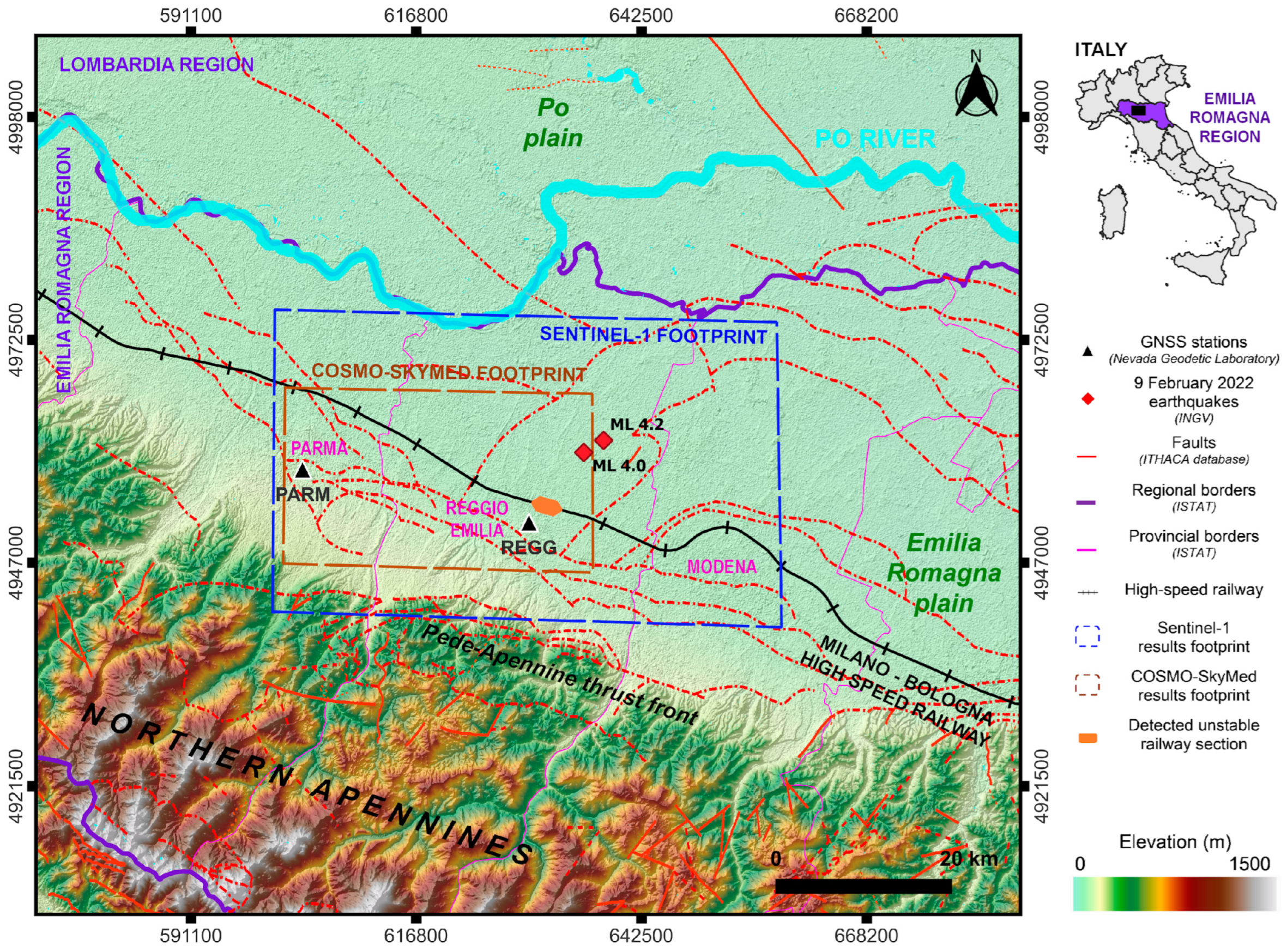The image is a detailed map primarily showcasing the Emilia-Romagna region in northern Italy, highlighted in purple. The map features various geographical and man-made elements, including a topographical representation with the northern Apennines mountains depicted in darker brown and yellow, and greener areas indicating lower elevations. Prominent on the map are several indicators such as GNSS stations, labeled by the Nevada Geodetic Laboratory, along with annotations marking the February 9, 2022 earthquakes, fault lines, regional and provincial borders, high-speed railway routes, Sentinel-1 and Cosmos SkyMed results footprints, and detected unstable railway sections. The key on the side provides further details, helping to identify the natural and infrastructural features, including river systems and the route network connecting cities like Parma, Modena, Milano, and Bologna. Overall, the map provides a comprehensive look at both the physical terrain and the critical infrastructure within the Emilia-Romagna region, reflecting impacts from seismic activity.